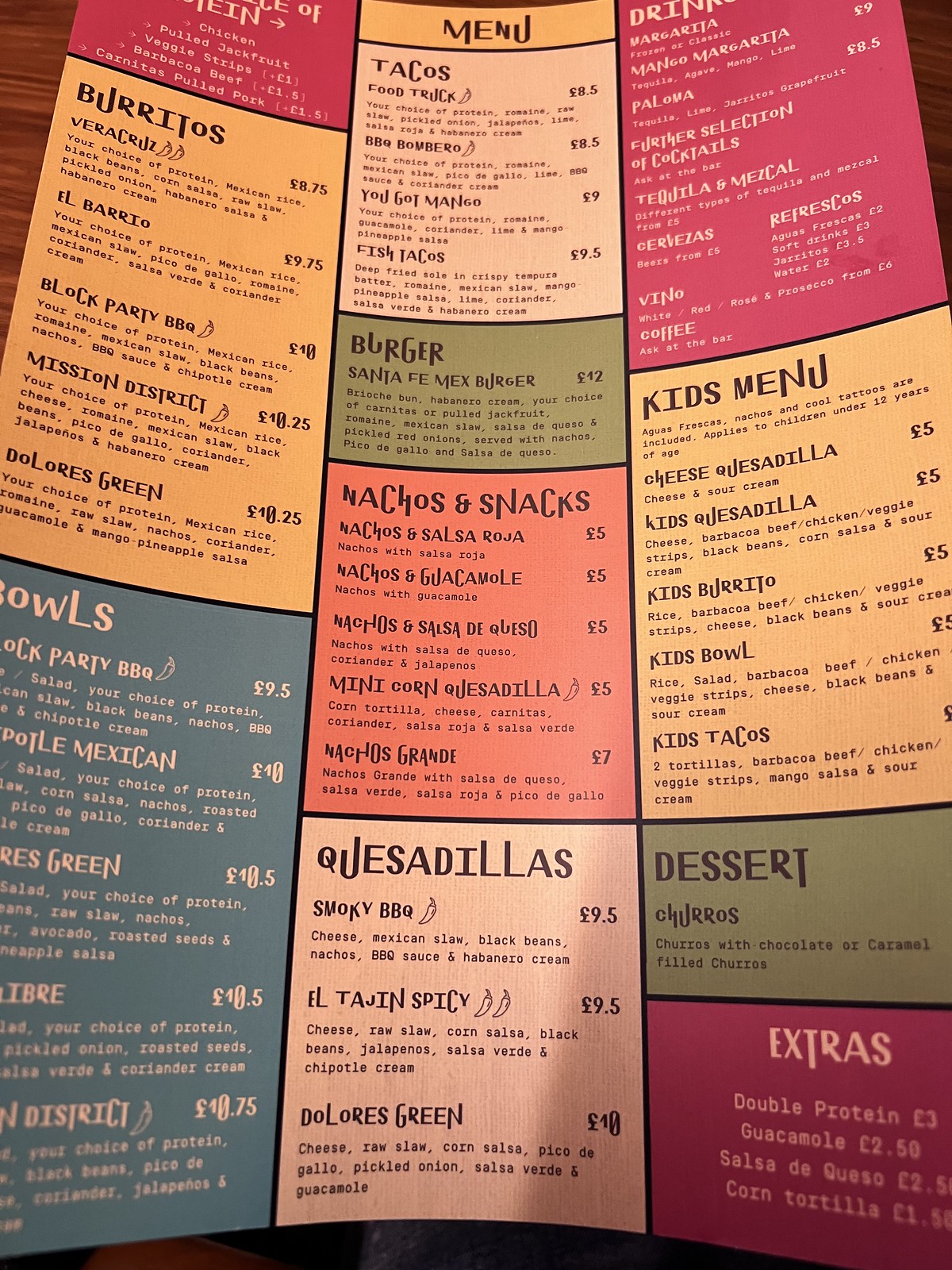This vibrant image features a kid's menu designed with a lively and colorful layout. The menu is segmented into various sections delineated by color-coded boxes, each representing different categories of dishes. The categories include Burritos, Tacos, Burgers, Kid's Specials, and Nacho Snacks. Each section offers a variety of options to choose from.

The color scheme consists of bright hues including blue, yellow, green, and teal, creating an eye-catching and inviting feel. The text displayed within these boxes alternates between white and black, depending on the background color, ensuring readability. This detailed and visually appealing layout is aimed at making meal selections fun and easy for young diners.